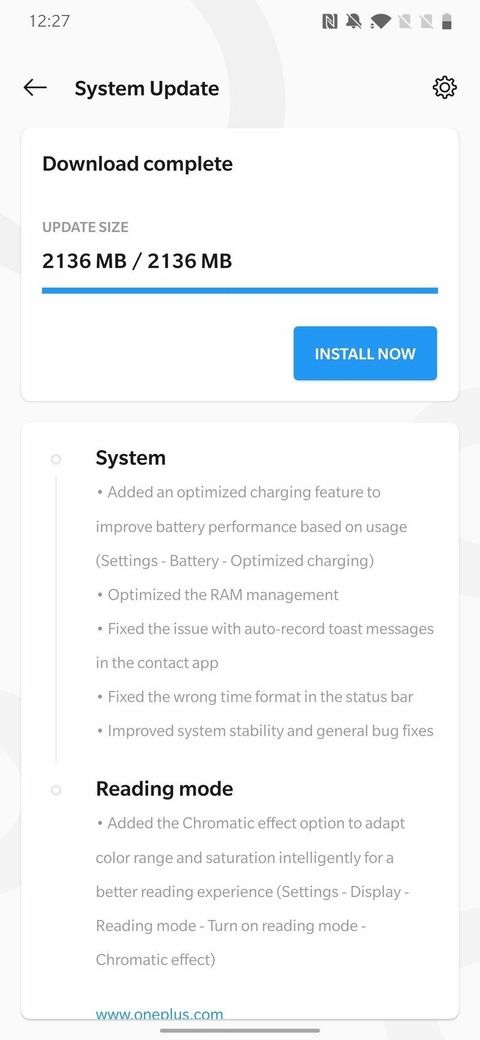Here is a clean and detailed caption for the image described:

---

The image is a screenshot of a smartphone display with a white background. Key indicators at the top-right corner confirm it's a phone: a notification bell, Wi-Fi signal, and a 50% battery icon are visible, along with a gear sprocket representing the settings. To the left of these icons, bold black text reads "System update" alongside a left-pointing arrow. The time in the top-left corner of the screen shows 12:27.

Below the "System update" heading, the text "Download complete" is prominently displayed in bold black. Following this, it indicates the update size as "2136 megabytes / 2136 megabytes," with a blue progress bar beneath this. Positioned to the right of the progress bar is a rectangular blue button labeled "Install now."

Further down, there are two paragraphs of information. The first is titled "System" and the second "Reading Mode." At the bottom of the screen, a light turquoise URL is displayed, reading "www.oneplus.com." The screenshot also captures part of a thick medium-gray bar located centrally, horizontally across the frame, though only partially visible.

---

This caption provides a clear, structured, and highly detailed description of the image contents.